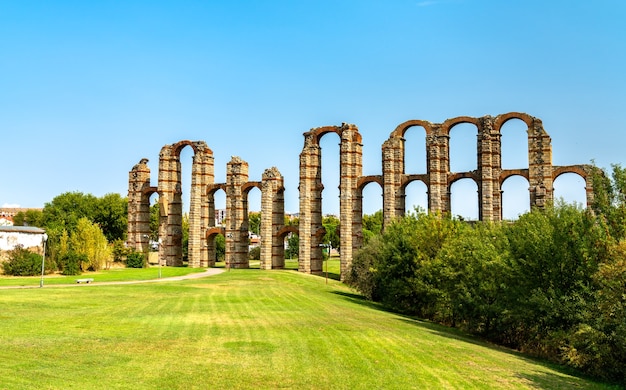The image captures a vibrant outdoor scene on a sunny day, featuring an eye-catching series of tall, interconnected arches made from light-colored beige bricks, evoking the feel of ancient ruins, possibly a Roman aqueduct. At least seven arches, varying in height and interwoven in an alternating pattern, stretch across the scene. The structure stands over a meticulously manicured, deep green lawn. A small, light gray road or pathway, dotted with lampposts and a bench, runs towards the arches and passes through one of them. On the right side of the image, there is a cluster of neatly trimmed green bushes, juxtaposing with more sizable bushes situated behind the arches. To the far left, a small gray building with a dark gray roof peeks out, partially obscured by additional greenery and a lamppost. The sky above is clear and blue, further enhancing the cheerful and serene ambiance of the landscape.